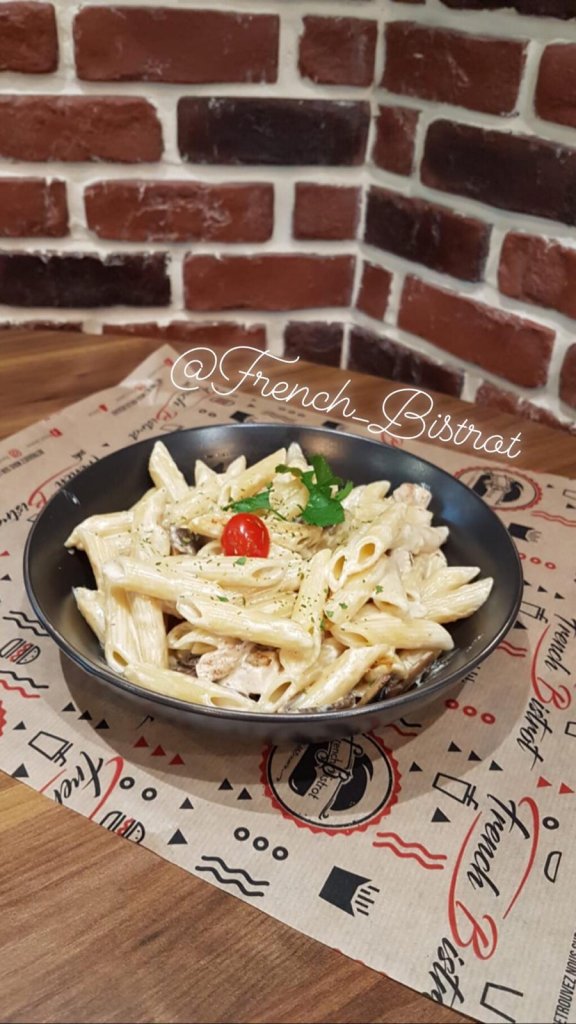In this detailed image, we are inside a restaurant suggested by the text "French Bistrot" in elegant white cursive on the brick walls in the background, spelled uniquely with a 'T' at the end. The walls are made of brick with white mortar, creating a warm, rustic ambiance. At the center of the image, on a wooden table, is a black ceramic bowl containing a pasta dish. The pasta appears to be penne, garnished with a single cherry tomato and some green leaves, possibly herbs, for flavor and aesthetic. The pasta is sprinkled with white cheese, possibly resembling fettuccine. The bowl is placed on a paper placemat featuring a pattern of red and black squiggly lines, circles, and triangles, adding a whimsical touch. The overall scene captures a snapshot of a restaurant's inviting atmosphere and a beautifully presented dish. There are no other people or objects present in the image.